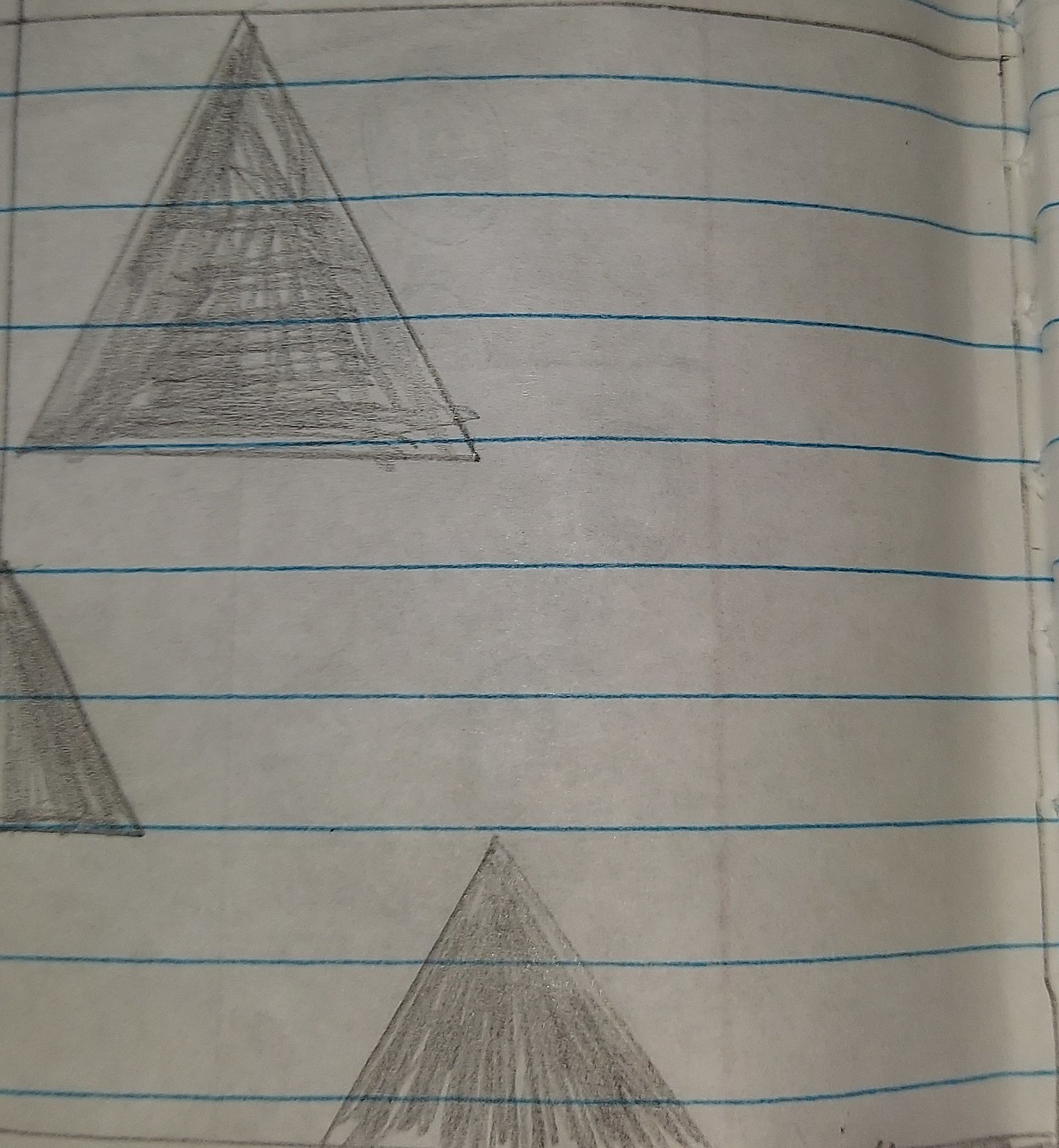The image features several hand-drawn triangles on traditional lined college-ruled notebook paper. The paper, characterized by its blue horizontal lines and a faint pink vertical margin on the right side, serves as the backdrop for the sketches. In the upper left-hand corner of the paper, there is a fully visible, equilateral triangle that has been shaded with scribbled pencil lines. Below this triangle, only the bottom right corner of another triangle is partially visible. At the very bottom of the image, there is the top portion of a third triangle, its complete shape cut off from view. The composition provides a casual, in-progress feel to the geometric sketches.